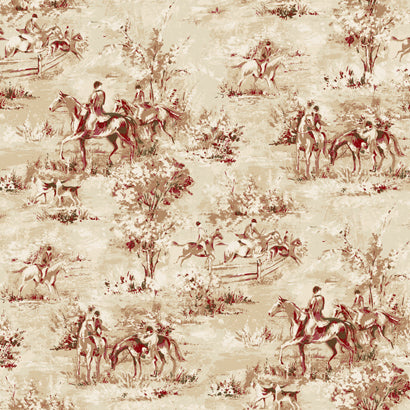This detailed illustration appears to be an old pen and ink drawing rendered in shades of brown, tan, and beige. It features multiple vignettes of English hunters and their horses, seamlessly tiled to form a cohesive yet repetitive pattern. The illustration includes several scenes: hunters on horseback, horses jumping over a fence, riders conversing, and a figure tending to a saddle. The artwork also depicts trees, shrubs, and hunting dogs. The figures and animals are not meticulously detailed but rather sketched in a more impressionistic style, contributing to the antiquated and artistic feel of the piece.